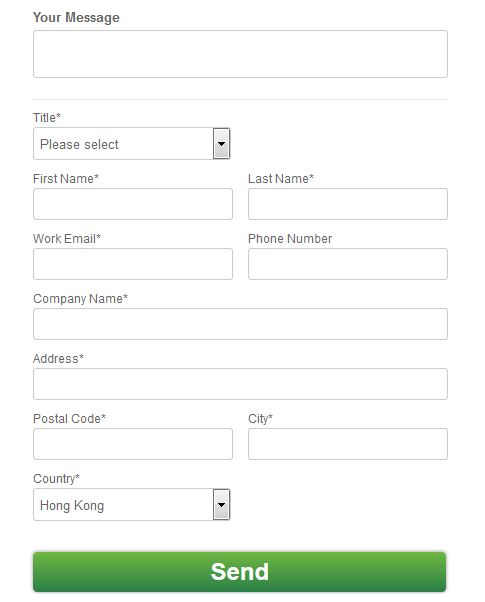Captured from a cell phone screen, this image showcases a detailed form layout with multiple interactive fields. At the top, a long blank rectangle is prominently labeled "Your Message." Below that, the "Title" field, marked with a required star, offers a drop-down menu for selection. Adjacent fields for "First Name" and "Last Name," both mandatory, are aligned on the same row. The subsequent row features the required "Work Email" and "Phone Number" fields. The "Company Name" field, also marked with a required star, occupies the next row entirely. Following this, two rows host fields for "Address," "Postal Code," "City," and "Country," each denoted with a mandatory star. At the bottom of the form, a green rectangular button with rounded edges spans the width of the screen, displaying the word "Send" in white print. The required fields stand out with a star symbol in their upper corners, indicating the necessity of completion.